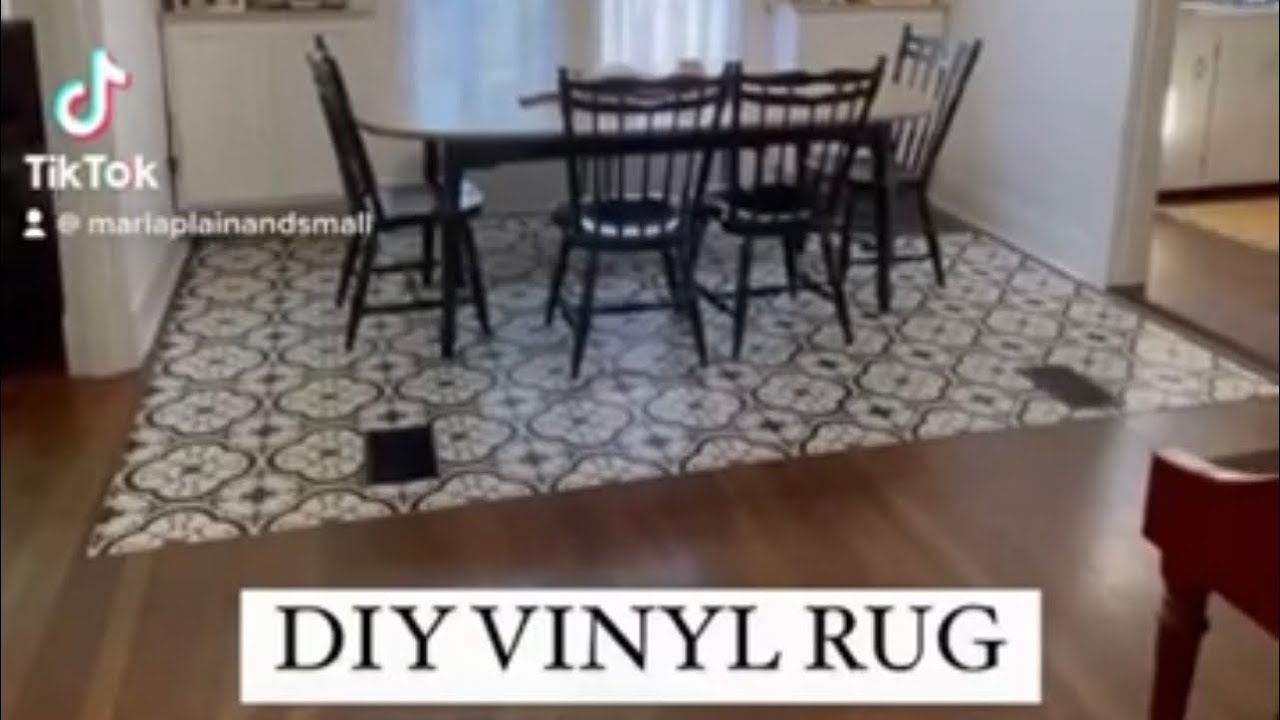This slightly out-of-focus image captures a cozy dining room, presented as a screenshot from TikTok by user Maria Plain and Small. The dining area features a black dining table with an oval shape, surrounded by four matching chairs—two of which face away from the viewer, while the other two are positioned on opposite sides. The set rests on a chic vinyl rug with a grey background and a prominent white floral pattern, inset within a larger, dark wooden floor. In the upper left corner of the image, the TikTok logo and user name are visible, while at the bottom, a white rectangle shows the text "DIY Vinyl Rug." The background reveals a window covered by a white curtain that lets in natural light. On the right side, there's a glimpse of additional furniture, possibly another table, contributing to the warm and inviting atmosphere of the interior. Two black rectangles, likely air vents, flank the patterned area nearer to the viewer, and there is an opening on the right side leading to another room, possibly the kitchen. The image emphasizes the stylish and practical homemade vinyl rug, showcased as a DIY project.